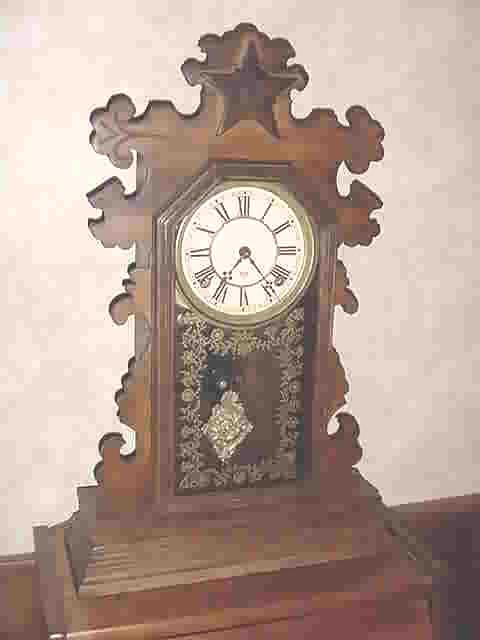This photograph captures a finely crafted wooden clock, slightly smaller in size compared to a traditional grandfather clock. The clock is made of orangey-brown wood and features intricate, ornate carvings throughout its design. Gold leaf work is visible just beneath the clock face, adding a touch of opulence. The clock face itself is a golden circle with an off-white background, adorned with Roman numerals instead of regular numbers. At the top of the clock, there is a beautifully carved wooden star. Surrounding the clock face, a series of leaf-like and more abstract wooden carvings add to its overall artistic appeal. The image quality becomes noticeably grainy and pixelated towards the bottom of the clock.